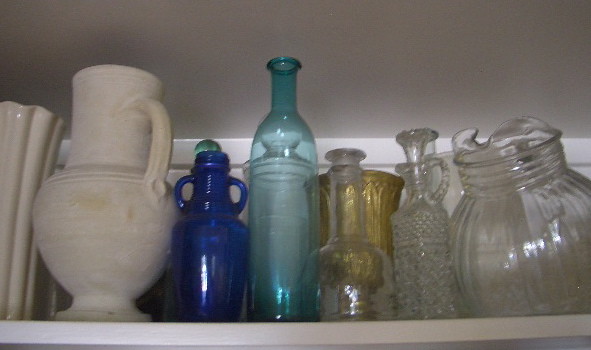This photograph captures the top shelf of a white cupboard, showcasing a diverse collection of approximately 15 vases and jugs. The shelf, placed close to the ceiling, is noticeably bowed under the weight of the glassware. The vases vary significantly in color, shape, and texture, suggesting a visually vibrant assembly. Among the collection, notable pieces include two blue glass vases—one turquoise and one cobalt—alongside several white vases with Greek and forest motifs. There is also a striking gold-painted vase and a variety of clear glass containers. Some items feature handles, reminiscent of pitchers, further adding to the assortment's eclectic nature. The arrangement appears haphazard, likely more for storage than display, with pieces pushed closely together, including a rounder vase on the right that seems precariously tipped. Overall, the collection is a colorful and textured ensemble against the uniform whiteness of the shelf and wall.